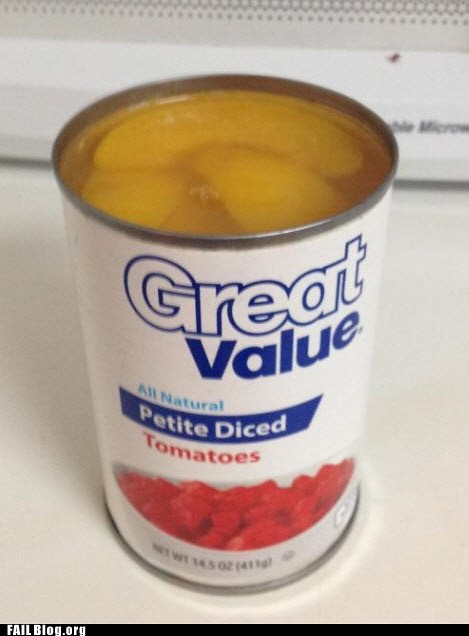This image features a small 14.5-ounce can typically used for tomatoes, but intriguingly, it contains peaches floating in juice. The can sports a white label prominently displaying the brand name "Great Value" at the top in large, bold letters, with "great" outlined in blue and "value" entirely in blue. Just below, the phrase "All Natural" appears in smaller letters. A blue box below that reads "Petite Diced Tomatoes," accompanied by a picture depicting small, neatly diced tomato pieces in a bowl. However, defying the label, the can's contents are actually peach slices immersed in their juice. The scene is set on a clean white counter with a white microwave visible in the background, adding a sense of everyday kitchen context.